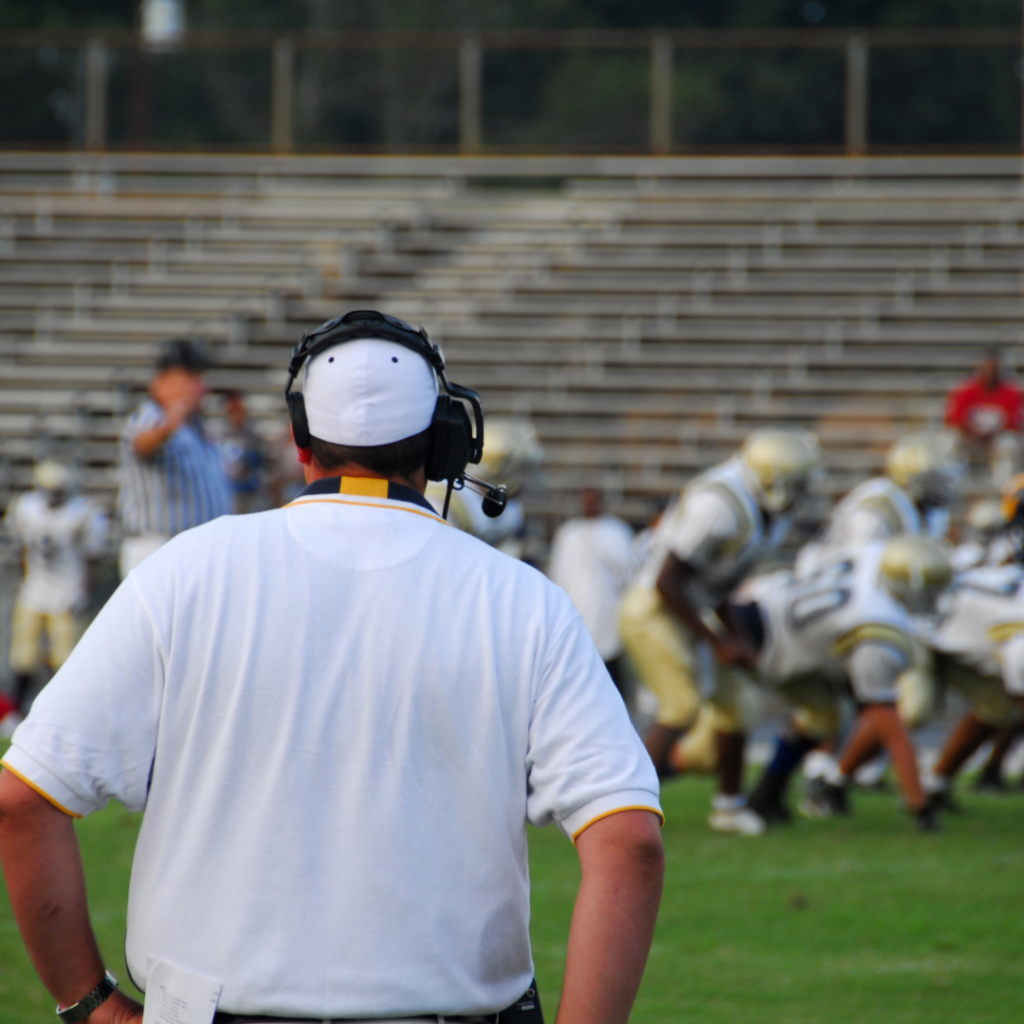In the foreground of this image, a coach stands with his back to the camera, wearing a white short-sleeved shirt with a blue and yellow collar peeking out. He has a white hat on his head, brown short hair, and a black headset with a microphone extending to the right side of his head. His hands rest on his hips, revealing a watch on his left wrist. The coach appears to be directing his attention towards the field, where a blurry football game is unfolding in the background. The players, difficult to distinguish, seem to be wearing gold helmets and gold leggings, and are positioned on the grassy field beneath the bleachers, which are empty. To the coach's left stands a referee, dressed in a striped black and white shirt and a black cap, with his arms raised as if signaling a timeout. The overall scene captures the dynamic environment of a football game, with clear emphasis on the coach's focused stance amidst the indistinct activity behind him.